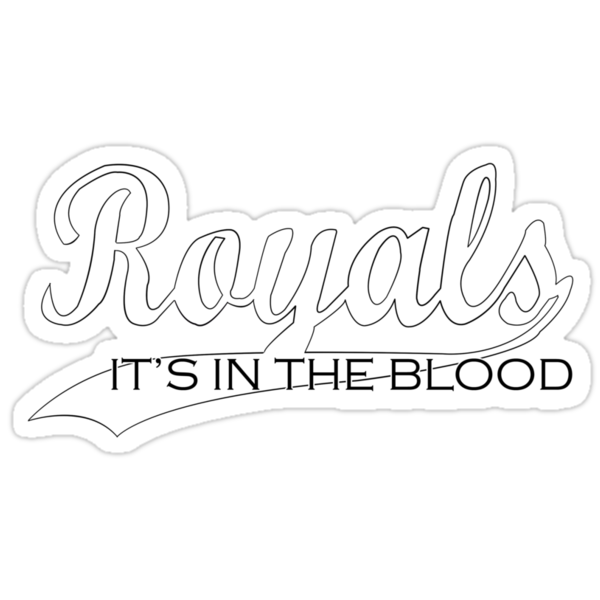The image is a detailed black and white template, potentially for a sticker or tattoo, featuring a bold, cursive logo of the word "ROYALS" in large bubble letters. The text is outlined with a light grey border that closely follows the shape of the letters. Extending from the end of the "S" in "ROYALS" is a long tail that underlines the word, creating a banner-like effect. Within this banner, in thin, bold print letters, it reads "it's in the blood." The entire design is monochromatic, with no shading or color, emphasizing its raw, outline format, suggesting it is meant as a template awaiting color or further detailing.